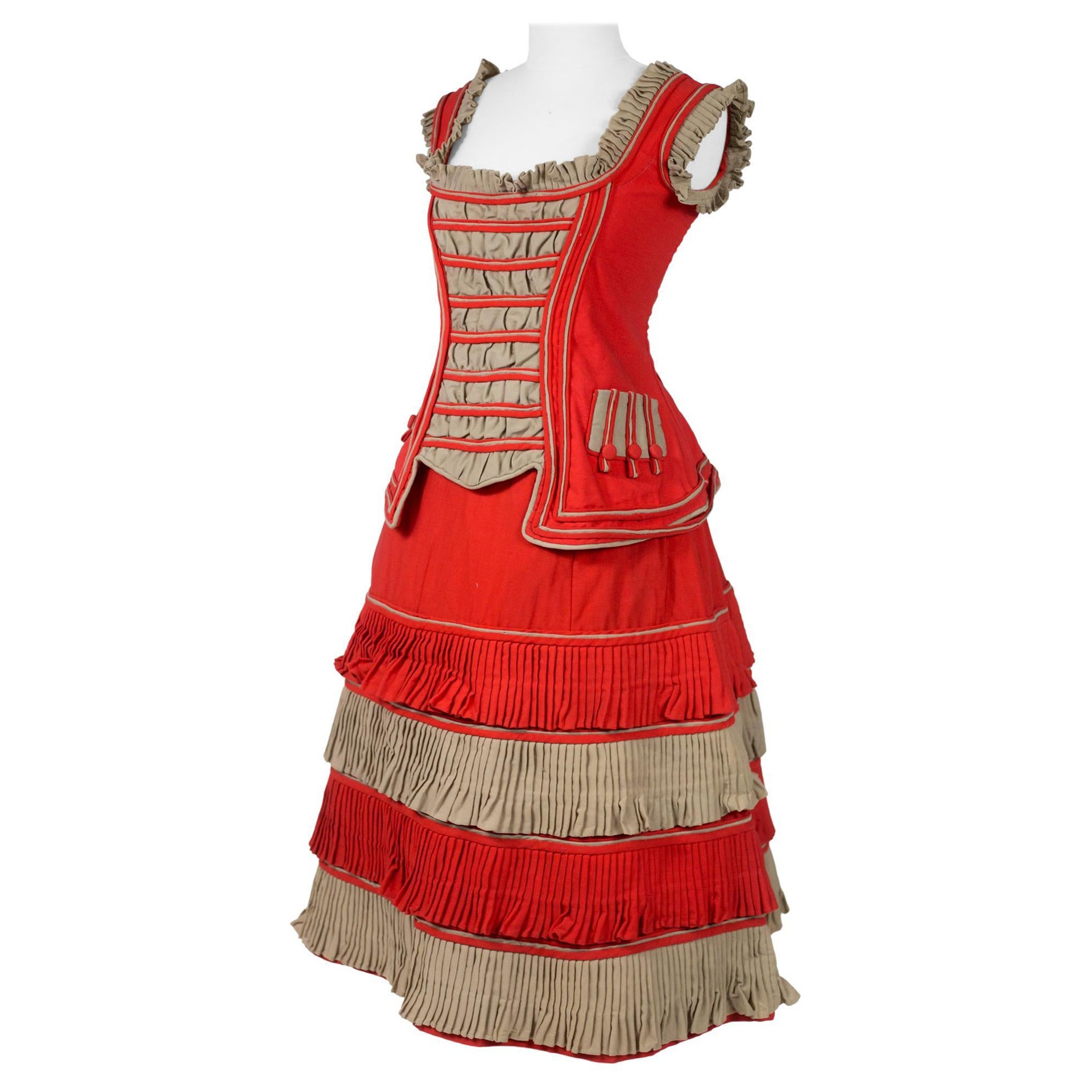This image features a headless and armless white mannequin dressed in an old-fashioned, museum-quality dress, set against a completely white background. The dress is a striking combination of muted red and dark beige, providing a richly detailed and historical appearance. The top of the dress includes a sleeveless bodice with gray ruffles adorning both the neckline and the shoulders. The neckline is square, revealing the upper chest area. The bodice itself is predominantly red with a central section of gray and red stripes, adding a visually textured element to the garment.

Moving down to the waist, the dress features a multi-layered, pleated skirt. The design alternates between red and gray pleats, starting with a solid red section at the hips, followed by a sequence of four distinct layered pleats: a red pleat, then a gray pleat, then another red, and finishing with a gray pleat at the bottom. Each pleated layer is accented with frills at the edges, contributing to both its visual and tactile richness.

The overall appearance of the dress, with its ruffled bodice and layered, frilled skirt, depicts an intricate blend of textures and colors that reflect a vintage, possibly regional European design.